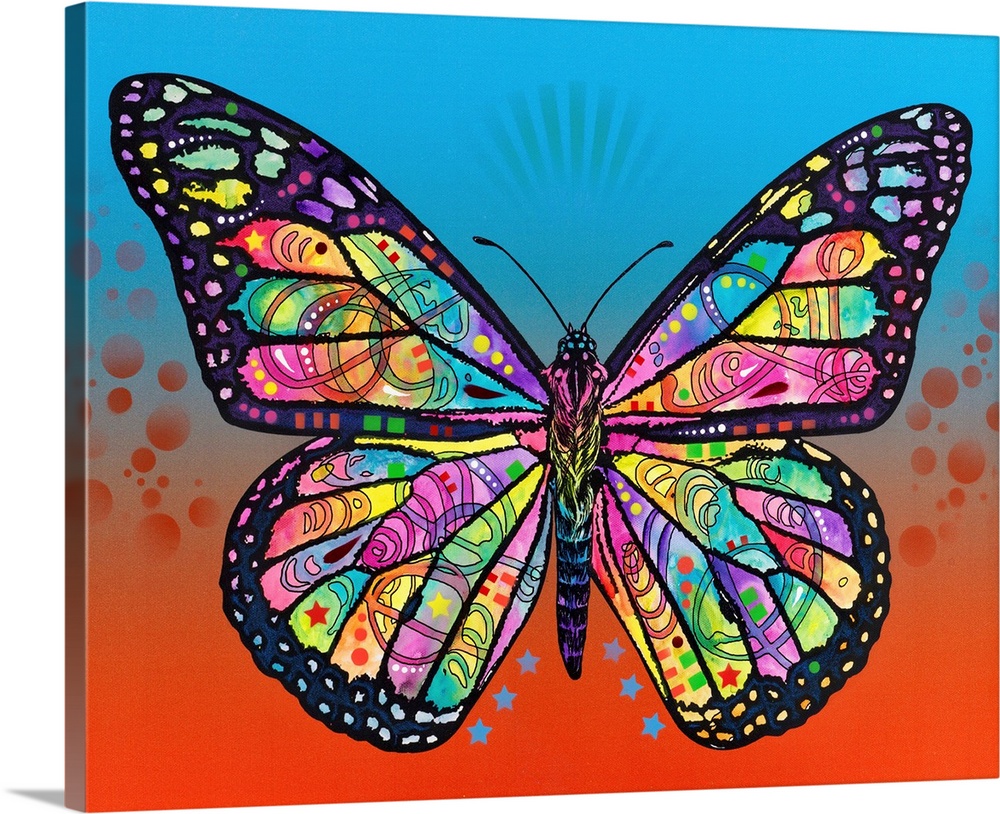This vibrant, computer-generated image depicts a fully spread butterfly seen from a top-down perspective, with its head facing upwards and its tail towards the bottom. The butterfly, outlined in a dark purple border almost black, exhibits a dazzling array of multicolored hues, including purples, blues, greens, yellows, reds, and pinks. Each wing features unique, asymmetrical designs with swirling patterns and colored dots, giving it a surreal, psychedelic quality.

The butterfly's body transitions through various colors, starting with a black-purple hue at the tail and changing to shades of blue-purple and yellow as it moves towards the head, which is notably black with pink and blue accents. Its black antennae are distinct against the colorful backdrop. The background of the image starts with a white color at the top and gradually fades into red towards the bottom, creating a sense of depth. There are red ball-like elements that seem to rise from the bottom, fading as they ascend. Additionally, three blue stars are positioned below the butterfly on either side, adding to the intricate details of the composition. The entire image has a 3D effect, with the edges of the canvas slightly curved and a faint shadow cast on the white background, enhancing its lifelike quality.